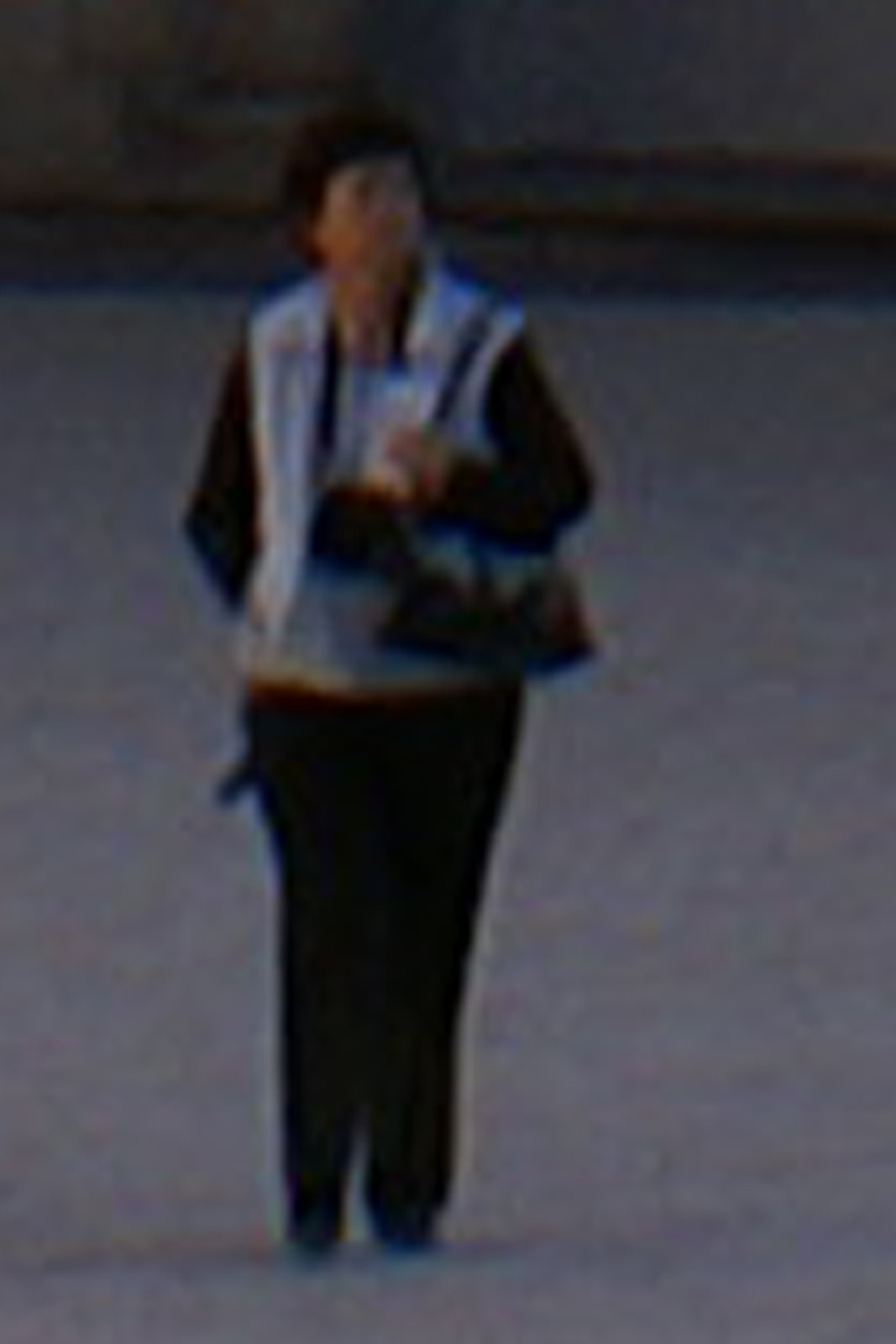A slightly blurred photograph, likely captured with a telephoto lens, depicts a middle-aged woman standing in what appears to be water or snow, as the lower part of her body and feet are obscured. She is dressed in black pants and a black long-sleeved shirt, complemented by a white vest. Over her left shoulder, she carries a handbag, which she is clutching with the same arm that also holds a plastic bag. The absence of an umbrella or hat suggests that any precipitation from above has ceased. She stands resolutely, possibly in a flood zone or an area affected by adverse weather conditions.